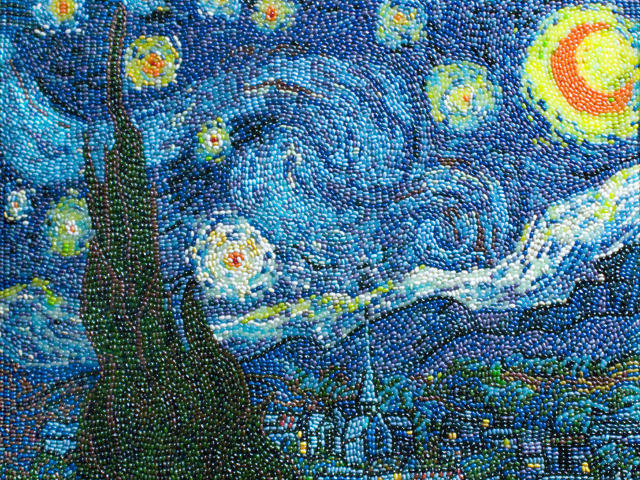This image is a textured, handmade rendition of Vincent van Gogh's famous painting, The Starry Night, created using colored beans or beads. The depiction closely imitates the original, with vivid, swirling shades of blue covering two-thirds of the scene to represent the night sky. The sky is adorned with scattered stars, circled in white, yellow, and orange, and features a crescent moon in a blend of darker orange and lighter yellow. The dynamic light blue swirl weaves through the sky, adding depth and movement. Below the celestial display lies a tranquil village with a chapel and distant mountains. A prominent, peculiar-looking green and brown tree stump or branch occupies the left forefront, adding an earthy contrast to the vibrant night sky.